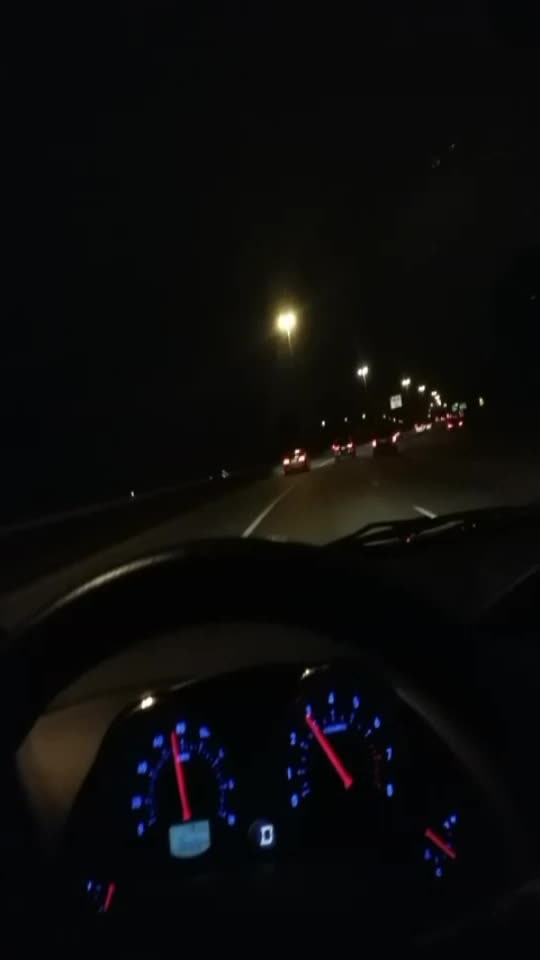This image captures the interior of a moving vehicle from the perspective of the driver's seat on the left-hand side. The dashboard and instrument panel are prominently displayed, featuring gauges illuminated in neon blue with red indicator needles. The steering wheel, dark in color, is positioned in front of the instrument panel, behind which part of the windshield wiper silhouette is visible. 

Through the windshield, several taillights from other vehicles are visible, suggesting the vehicle is navigating a four-lane road. The car is positioned in the second lane from the left, separated by a solid white line from the leftmost lane. The adjacent lane to the right is demarcated by a dashed white line. Overhead, street lamps light up the road ahead, providing additional context to the nighttime driving scene.